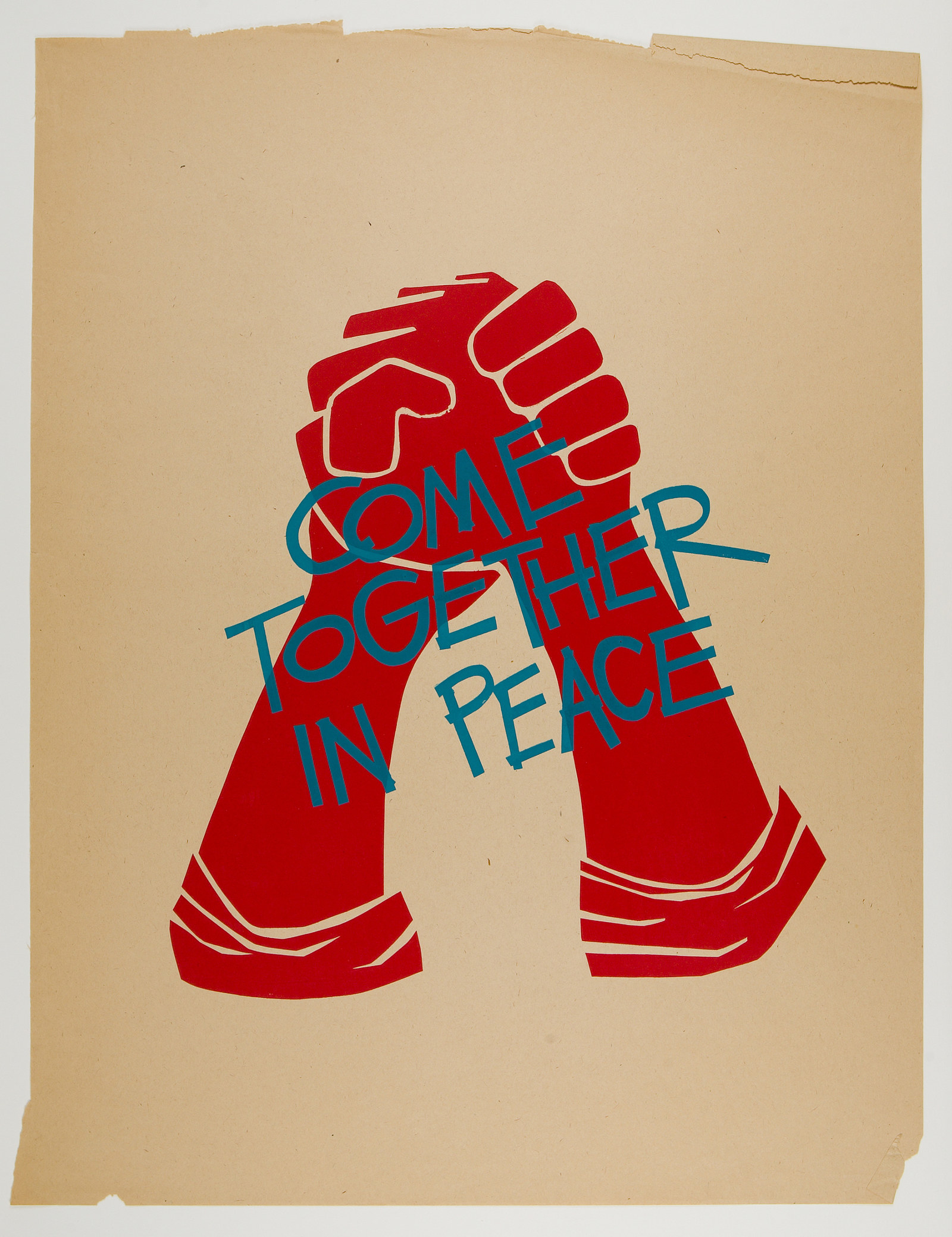The image is a rectangular poster with a taller height compared to its width, featuring an off-white or light gray background. Layered on top is a slightly worn, ripped, and folded piece of manila or beige-peach toned paper, suggesting it has been used or displayed multiple times. The focal point of the poster is the message in large, blue, capital letters that reads "COME TOGETHER IN PEACE," arranged slightly diagonally, descending from left to right. Below this text, two red hands, extending to elbows and depicted in a graphic, cartoon-like style, are clasped together, symbolizing unity and support. The image captures a sense of aged, heartfelt appeal, with its worn edges and visible textures.